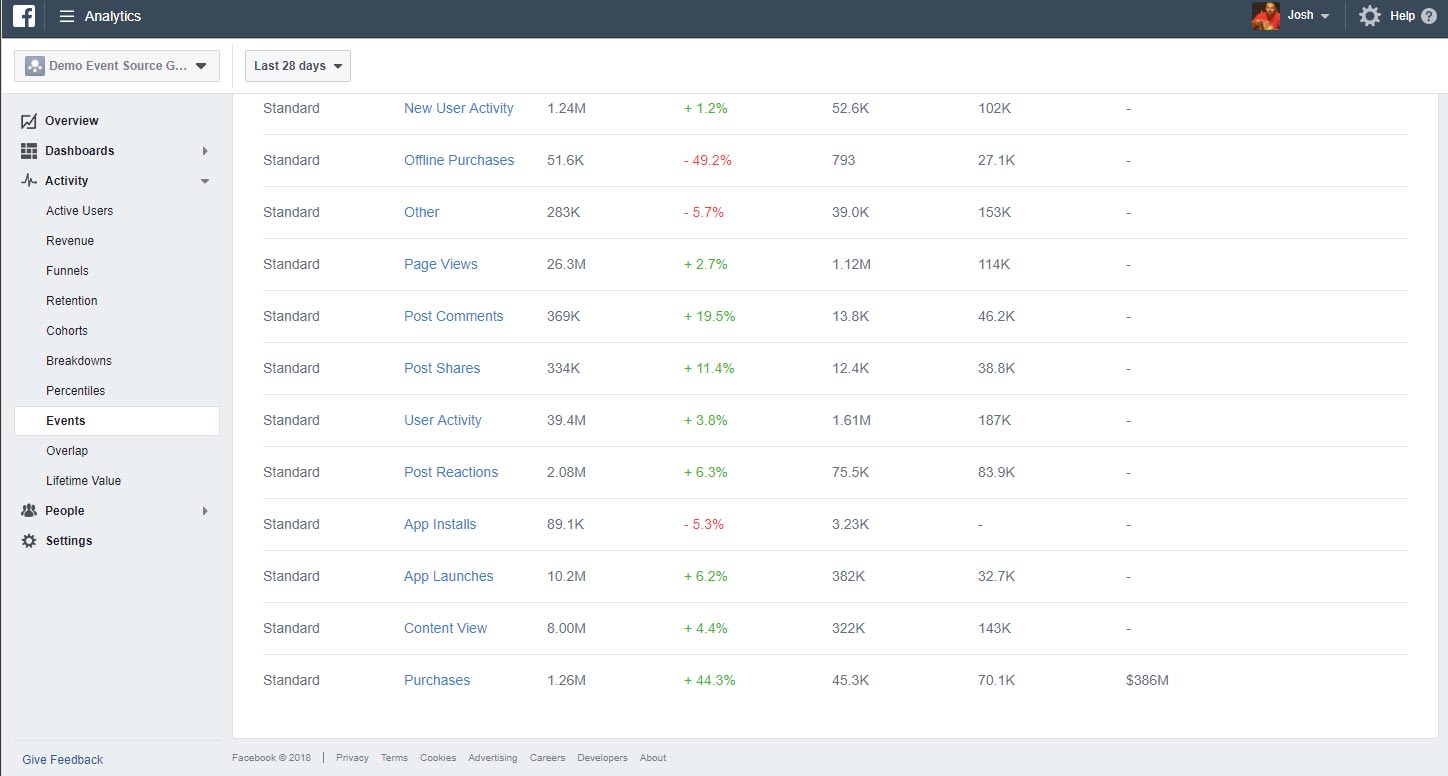The image appears to be a screenshot likely taken from someone's Facebook or Facebook Marketplace account, given the identifiable 'F' icon in the upper left-hand corner. In the upper right-hand corner, there is a profile picture, perhaps belonging to a user named Josh. The dashboard displays various analytics, with a prominent text ‘Last 28 days’ indicating a specific time frame for the data presented. On the left-hand side of the screen, there is a light blue navigation column displaying menu options such as 'Overview,' 'Dashboard Activity,' 'Active Users,' and possibly 'Events' or another related term that isn't fully legible. Within the analytics, numbers like 1.24 million for new user activity and a green +1.2% indicate user growth, while figures like 52.6K and 102K suggest different metrics or benchmarks being tracked. The overall layout and statistics resemble a performance or activity report commonly used for tracking user interaction and engagement on social platforms.